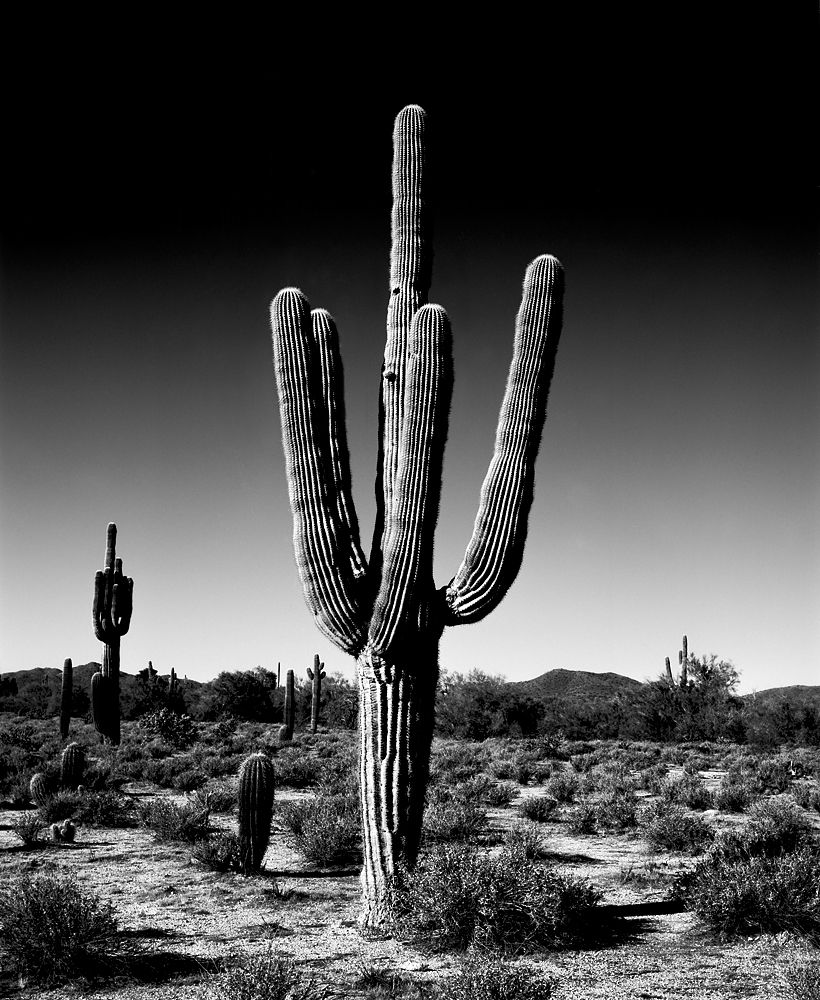This striking black and white photograph captures a picturesque cactus landscape bathed in contrasting shades of gray. Dominating the center of the image is a majestic saguaro cactus, with a tall central stem flanked by four extended arms curving gently before rising skyward. The desert floor at its base is adorned with scattered tumbleweeds and small bushes, contributing to the sparse yet rugged terrain. To the left, a smaller, pickle-shaped cactus and various other single-stemmed cacti of different heights punctuate the scene. Further back, several more tall cacti with upward-reaching arms can be seen. The rolling hills or mountains form a distant backdrop, adding depth to the composition. The sky transitions from a light gray near the horizon to a darker gray, eventually fading to black at the top, casting elongated shadows across the ground and enhancing the dramatic atmosphere of this serene desert vista.